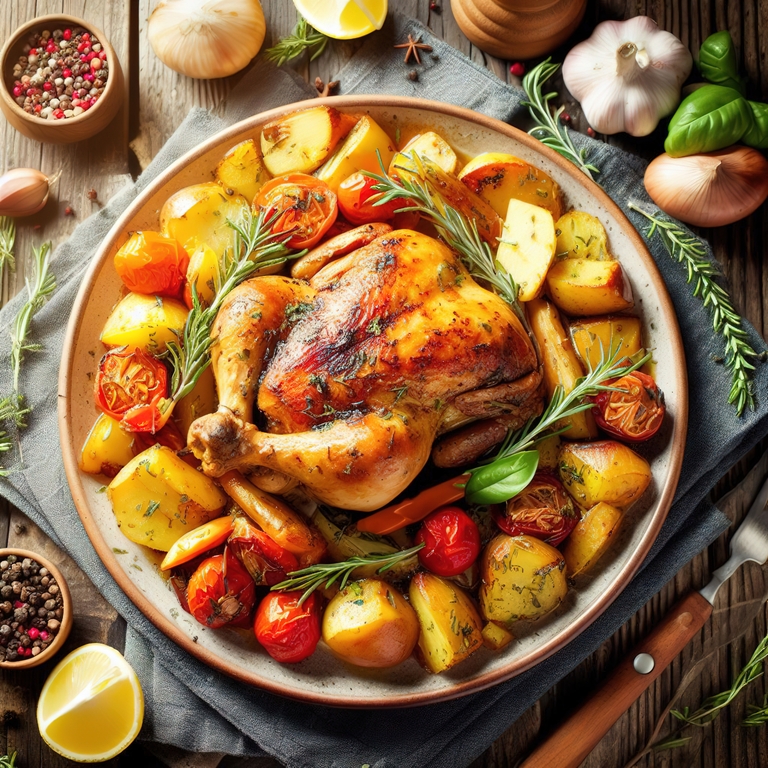A mouthwatering cooked meal takes center stage on a large dish, featuring a perfectly roasted Cornish hen or chicken. The succulent bird is garnished with fragrant sprigs of rosemary, accompanied by a medley of golden roasted potatoes and vibrant red tomatoes. Additional rosemary encircles the dish, with a solitary basil leaf hidden beneath the bird, adding a burst of green. The meal is presented in a bowl adorned with a brown trim and a beige interior, set on a gray napkin that is meticulously placed in a diamond shape. Scattered on the napkin are a few fresh basil leaves, complementing the rustic aesthetic.

In the upper frame, a fork partially enters from the bottom right corner, its handle crafted from brown wood and its tines glistening silver. Various herbs and spices, including onions, garlic cloves, and what appears to be star anise, are thoughtfully arranged around the scene. On the left, a small container of red, brown, and beige spices mingles with additional garlic cloves and a lemon wedge. More sprigs of rosemary peek in from the lower right-hand side, completing the harmonious display on what seems to be a wooden table.

This meticulously arranged setting effortlessly blends colors and textures, inviting viewers to savor the sensory delight of a beautifully prepared meal.